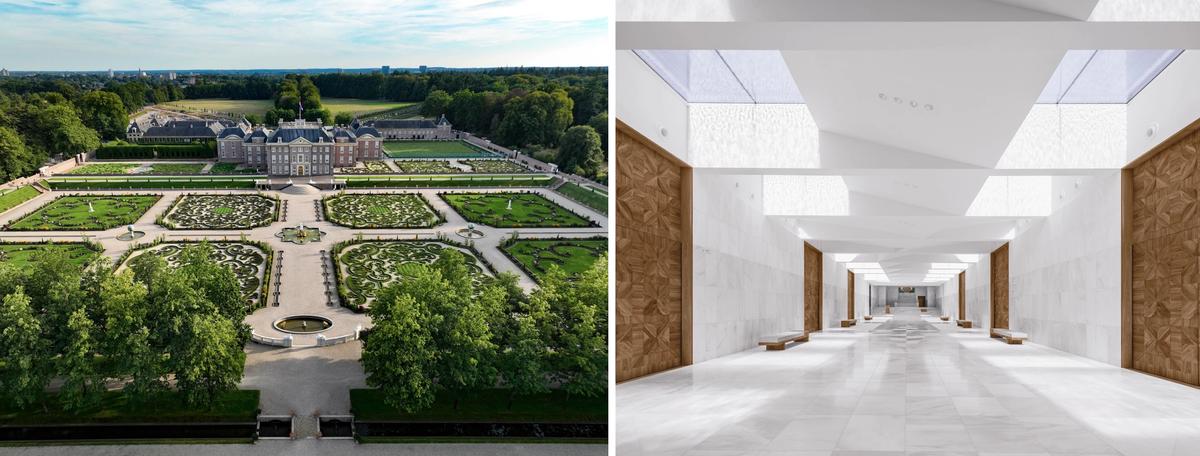The image features a side-by-side display of two different photos. On the left, an expansive, elevated photo captures a picturesque estate with a blue sky above. The estate is a castle-like mansion, comprising three or four stories with tiered sections that step back incrementally. The lush grounds are meticulously designed with a large garden, featuring a grid of walkways and neat garden plots. There are fountains strategically placed at the intersections of these walkways, surrounded by various trees and greenery, enhancing the serenity of the courtyard.

On the right, the interior of the mansion is showcased, revealing a long, minimalist corridor bathed in natural light from skylights embedded in the ceiling. This corridor, predominantly adorned with white marble, features evenly spaced wooden panels resembling large doors along the walls. Between these panels are low benches that are a combination of white and brown marble, contributing to the clean and sophisticated aesthetic of the space. The pristine and uncluttered appearance of the hallway emphasizes the grandeur and serene ambiance of the mansion's interior.